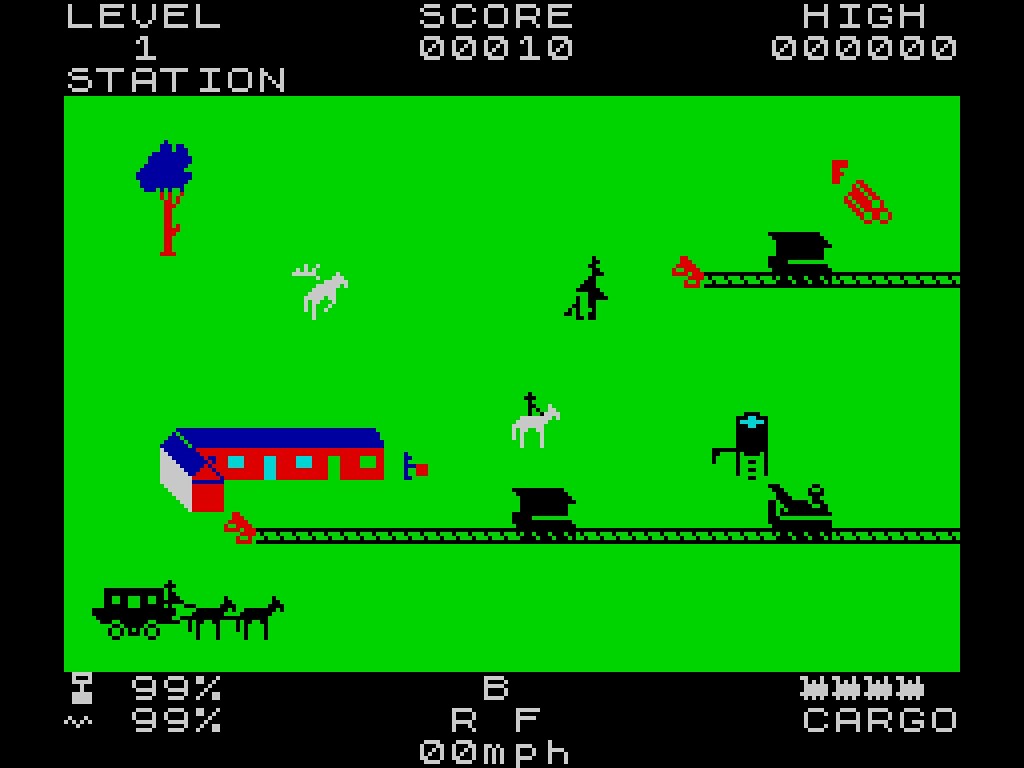The video game display features a vivid lime green background, upon which rests an intricate network of black railways and train carts. In the foreground, a silhouetted horse and carriage add a touch of classic charm. To the right, a striking pink building with a purple roof stands prominently, accompanied by white horses scattered around its vicinity. The entire scene is framed by black VIC borders, giving it a distinct, retro appearance. At the top left corner, white text boldly declares "LEVEL 1 STATION." Additional text overlays include a score of 10, a high score of 0, and the word "CARGO" in the bottom right corner, providing essential game information.